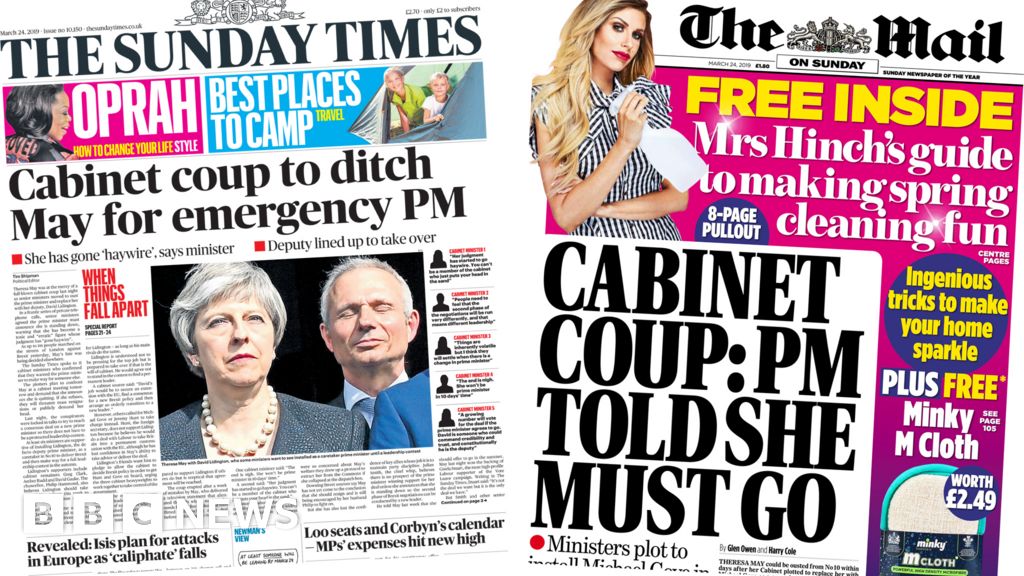The image displays the covers of two newspapers side-by-side. 

On the left, the front page is from "The Sunday Times." The header is primarily blue. Below the title, there's a prominent pink rectangle housing the headline "Oprah" in white, discussing how she can help change your life, accompanied by "Telling Society Oprah" in smaller text. Below this, a blue rectangle features the headline "Best Places to Camp" in white, and a yellow rectangle underneath highlights "Travel with Two Kids" over an image of two children emerging from a tent. There is a white background with black text stating "Cabinet coup to ditch May for emergency PM," followed by the phrase "She has gone haywire" attributed to a minister, and mentioning a deputy lined up to take over. Another section says, "When Things Fall Apart — Special Report" in black, possibly spanning pages 27 or 21 to 30-something. Towards the bottom, "Revealed" in black letters details ISIS plans for attacks as Europe's caliphate falls, mentioning loose seats and "Corbyn's Canada." Finally, it says, "MPs expenses at new high" in white letters on a black background, accompanied by the CBBC News logo.

On the right, the other cover is from "The Mail on Sunday." The headline in yellow states "Free Inside," with a subheader in white that reads, "A Mrs. Hinch Guide to Spring Clean & Shine." In black letters, it states, "Cabinet PM Told She Must Go," likely referring to the Prime Minister. Additionally, a purple section in white text offers "Ingenious Tricks to Make Your Home Sparkle" and highlights a "Free Minky & Cloth" offer.